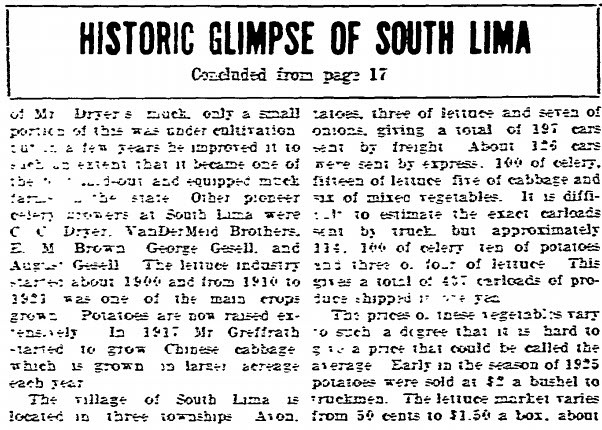The image features an old, black-and-white newspaper article titled "Historic Glimpse of South Lima," enclosed in a black rectangular box at the top. The article, continued from page 17, is printed with type that is faded and partially missing, making it difficult to read. The layout includes two columns of text, a common format in vintage magazines. The left column mentions Mr. Dreyer and the agricultural conditions of 1925, including details about potatoes being sold at $2 a bushel to truckmen and lettuce at prices ranging from $0.50 to $2.50 a box. It also highlights the village of South Lima, located within three townships. Another pioneer, George, and Mr. Griffith are noted, with references to the lettuce industry and extensive potato farming. The right column contains additional paragraphs, equally as worn and challenging to decipher. Overall, the article offers a fragmented yet intriguing glimpse into the agricultural history and community of South Lima.